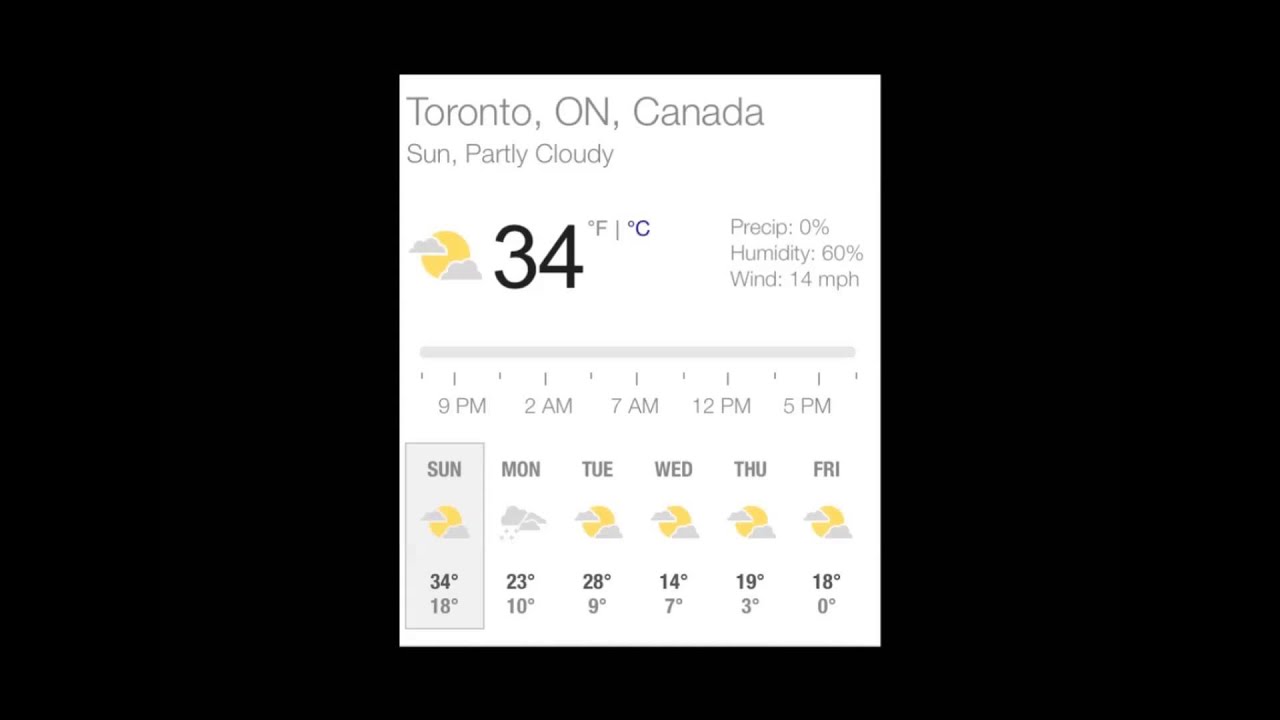The image features a black background with a white rectangle centered in the middle. In the upper-left corner of this white rectangle, the text "Toronto, Ontario, Canada" is displayed. Below that, it reads "Sun, partly cloudy," accompanied by a sun and a couple of clouds.

Prominently displayed is the temperature: "34°C" in large, black text, which is emphasized by a highlighted backdrop. On the right side of the white rectangle, there is information about the weather conditions: "Precipitation 0%," "Humidity 60%," and "Wind 14 miles/hour."

Beneath this main section, a gray horizontal bar divides the rectangle. Below this bar, the times "9 p.m., 2 a.m., 7 a.m., 12 p.m., and 5 p.m." are listed. Further down, the days of the week from Sunday to Friday are indicated, each with their respective weather icons and temperatures.

For Sunday, there is an icon of the sun and clouds, with a high of 34°C and a low of 18°C. Monday shows a cloud with raindrops, with temperatures of 23°C for the high and 10°C for the low. Tuesday is represented by the sun and clouds again, with a high of 28°C and a low of 9°C. 

Wednesday through Friday consistently show a sun and clouds icon. Wednesday has a high of 14°C and a low of 7°C. Thursday's temperature peaks at 19°C with a low of 3°C, and Friday rounds out the week with a high of 18°C and a low of 0°C.